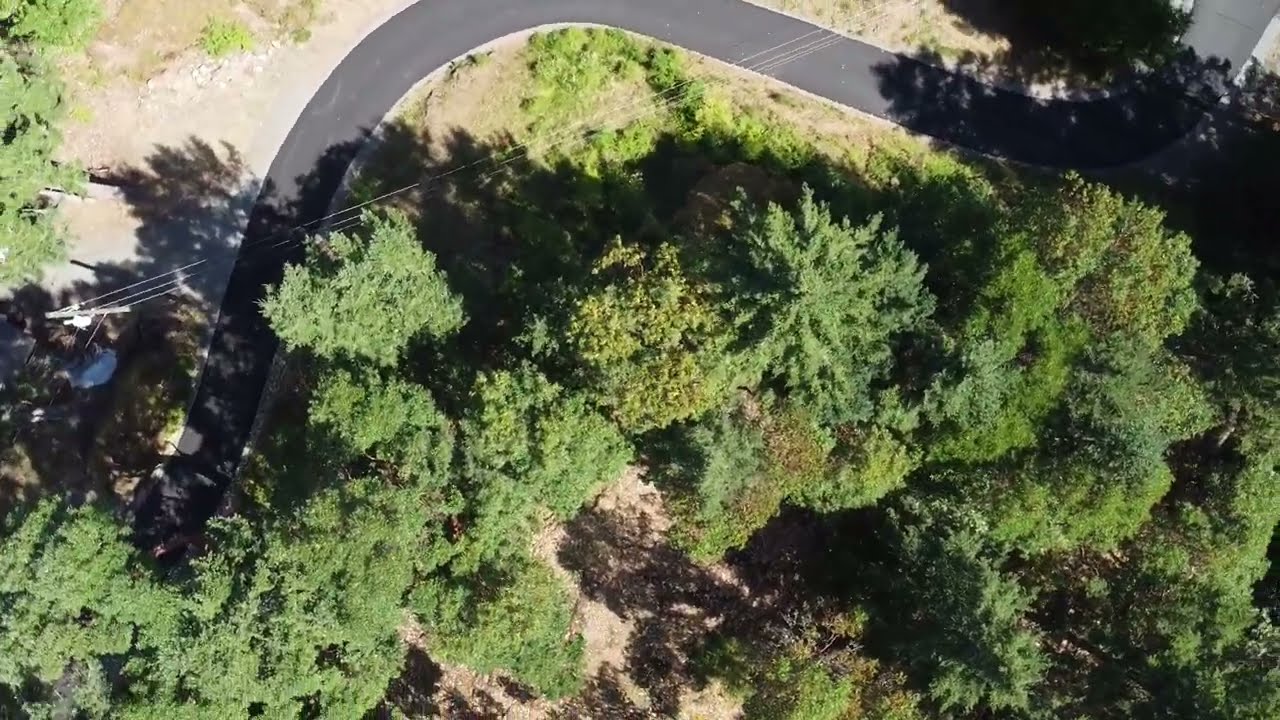An overhead view captured by a drone during the daytime showcases a vibrant, natural landscape. The image is in color with high clarity, allowing for an appreciation of the bright green hue of the large trees occupying the lower portion of the photograph. The main feature is a winding, dark gray path that begins at the top right corner and snake-like, moves towards the bottom left, fading into the dense forested area. The path, likely a walking trail, is bordered by patches of light beige dirt and grass. The scene is devoid of any people, vehicles, letters, or numbers, emphasizing the solitude and natural beauty of the area. Additionally, tree shadows can be seen adding depth to the landscape, and a small building is situated near the bottom left center of the image. The outdoor setting is illuminated by abundant natural light, indicative of a bright, clear day.